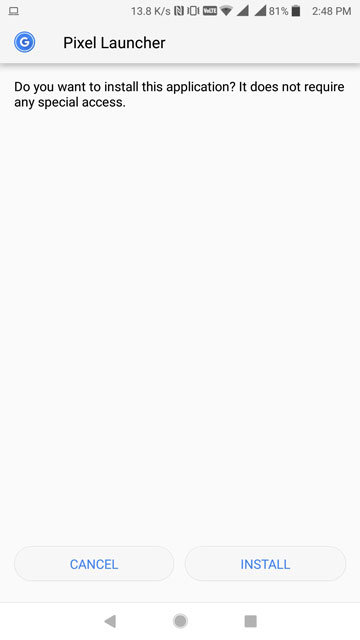A detailed cell phone screenshot taken at 2:48 p.m. reveals various elements on the screen. The phone's battery is at 81%, and it has full network coverage with four bars, as well as three out of four bars on the Wi-Fi network. The phone is in vibrate mode and is identified as a Voltaire or Vortex, a government-provided device with a connection speed of 13.8 kilobytes per second. An icon of a computer monitor and keyboard appears in the upper-left corner of the screen.

Below the top status bar, the screen displays "Pixel Launcher" in black letters, accompanied by a blue circle with a white "G" in the center, which is presumably the icon for the Pixel Launcher app. Further down, a prompt reads, "Do you want to install this application?" followed by a note stating, "It does not require any special access." This text is presented in black letters.

At the bottom of this prompt are two buttons: "Cancel" and "Install," both in blue letters inside oblong buttons. The very bottom of the screen features the standard navigation buttons found on most cell phones: a triangle for going back, a circle for returning to the home screen, and a square for toggling between open applications.